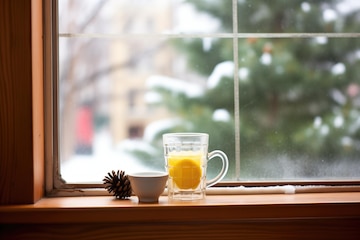The photo is a close-up, colored still life of a well-polished wooden windowsill adorned with a few detailed objects. Positioned on the left, a tiny pine cone sits beside a small white teacup, and to their right, a clear glass mug with a yellow ball or fruit inside, possibly orange juice. The window frame shows only the left and bottom parts, exhibiting white trim and a slightly visible wooden pillar with metal elements and caulking at the corners. Outside the blurred, cross-etched window, a snowy scene reveals a towering pine tree dusted with snow and a distant multi-story barn-like building.